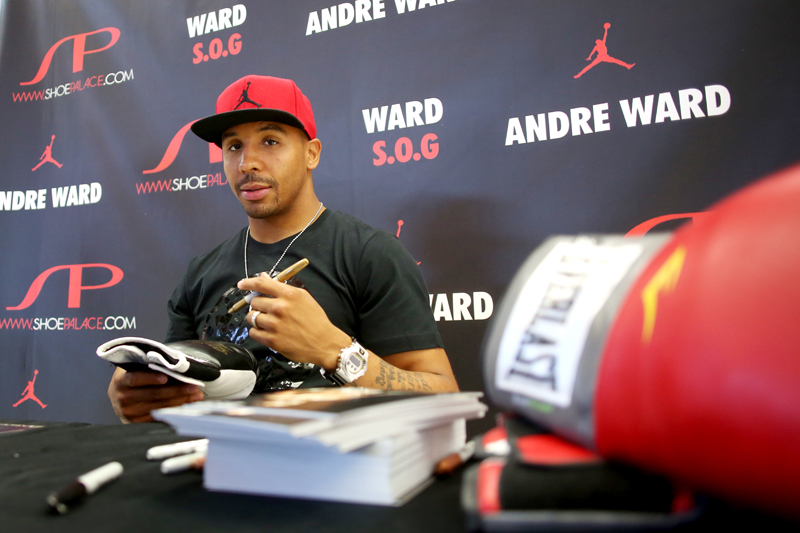The image features Andre Ward sitting behind a desk or podium, engaged in a signing session. The background is a black banner adorned with multiple rows of text reading "www.shoepalace.com," "Ward SOG," and "Andre Ward." Andre, identifiable by the signage, is wearing a red Nike Air Jordan cap, a black t-shirt, and a visible chain necklace. In his left hand, he holds a marker while his right hand holds a black boxing glove, which he is about to sign. In front of him, there are stacks of books and another Everlast boxing glove on the right side of the table.